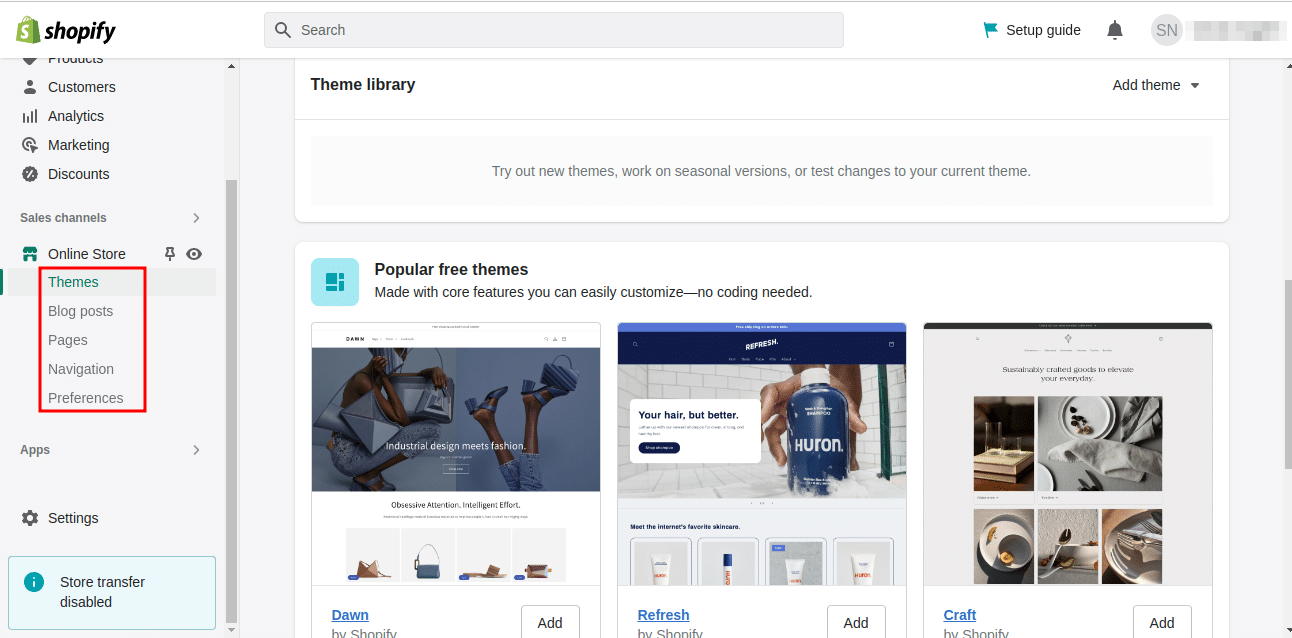This image depicts a web page titled 'Theme Library,' promoting new and customizable themes for seasonal updates or testing changes to current themes without requiring any coding skills. 

Under a prominent heading that reads, "Popular Free Themes Made with Core Features You Can Easily Customize, No Coding Required," multiple visual elements make up the content.

Starting from the left, there is a section titled "Dorm by Shoofi," featuring items such as handbags. A notice on this section states, "Store Transfer Disabled," which may suggest limited functionality.

In the center of the webpage, various toiletries are displayed neatly within a narrow slot. A notable middle section displays a bottle with the label "Huron, Your Hair But Better."

To the right of this, there are smaller images. One resembles a bed, another shows towels, and there appears to be an image of a serving dish. Additional images, though not clearly identifiable, hint at a variety of cozy or luxurious items.

Adding to the luxurious theme, there is also a picture of someone sitting in a spa with their feet elevated, and another individual is seen squatting near a poolside, wrapped in a towel, likely in a sauna or similar relaxation setting. 

Overall, the web page aims to entice users with its variety of customizable, feature-rich themes showcased next to lifestyle imagery suggestive of comfort and luxury.